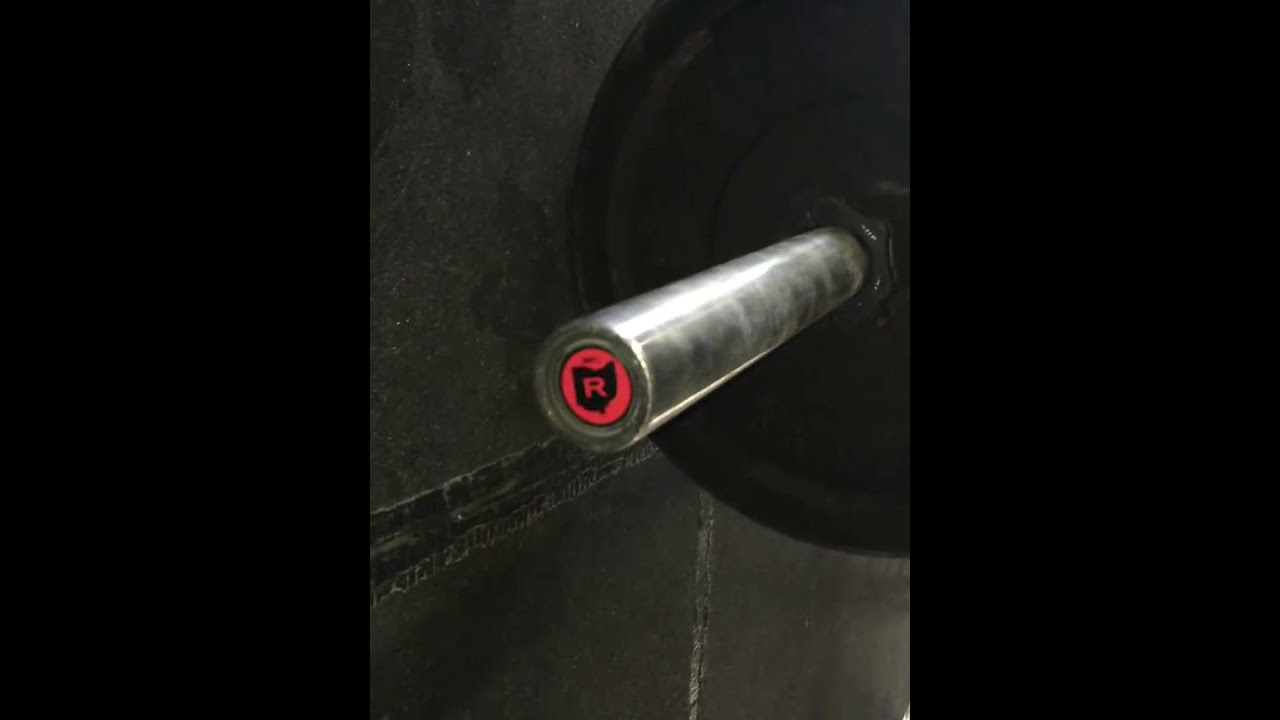This image features a dark, primarily black and gray background resembling a cement or possibly metal surface, suggesting it might be a garage or gym. At the center of the image, there's a metallic silver pole protruding from a black circular object, with a red circular ornament at the end marked with the letter "R." The scene is minimalistic with the primary colors being black, gray, silver, red, and hints of white. The environment appears utilitarian, possibly for weightlifting or similar activities, though the exact nature of the objects remains ambiguous.